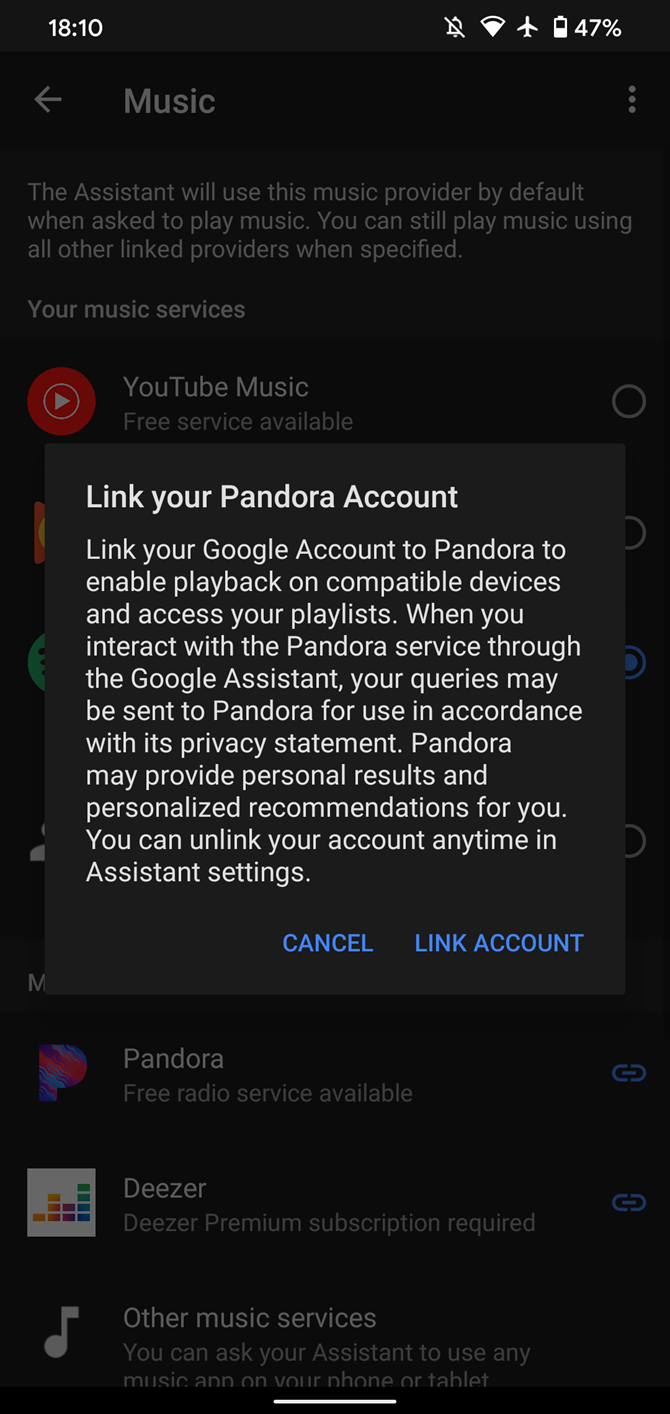This is a detailed and cleaned-up descriptive caption for the screenshot provided:

---

In this screenshot taken at 18:10 military time, the phone's notifications are disabled, Wi-Fi signal is nearly full, and Airplane Mode is activated. The battery level is at 47%. The screen is darkened, and the phone is currently in the Music menu. The interface indicates that the Google Assistant is set as the default music provider, able to play music from various linked services when specified. 

The YouTube Music app is currently highlighted, with a prominent black box prompt suggesting the user to link their Pandora account to Google. The message advises that linking the Pandora account will enable music playback on compatible devices and provide access to personalized playlists. It also mentions that queries to Pandora through the Google Assistant may be sent to Pandora and could yield personalized recommendations based on their privacy statement. Users are informed they can unlink their account at any time via the Assistant settings, with clear, blue buttons for "Cancel" and "Link Account."

Behind the prompt, the application interface hints at requiring a premium subscription for full access. The overall appearance notes that there is no option for playing unlicensed or pirated music on this phone, emphasizing the use of legitimate service links only.